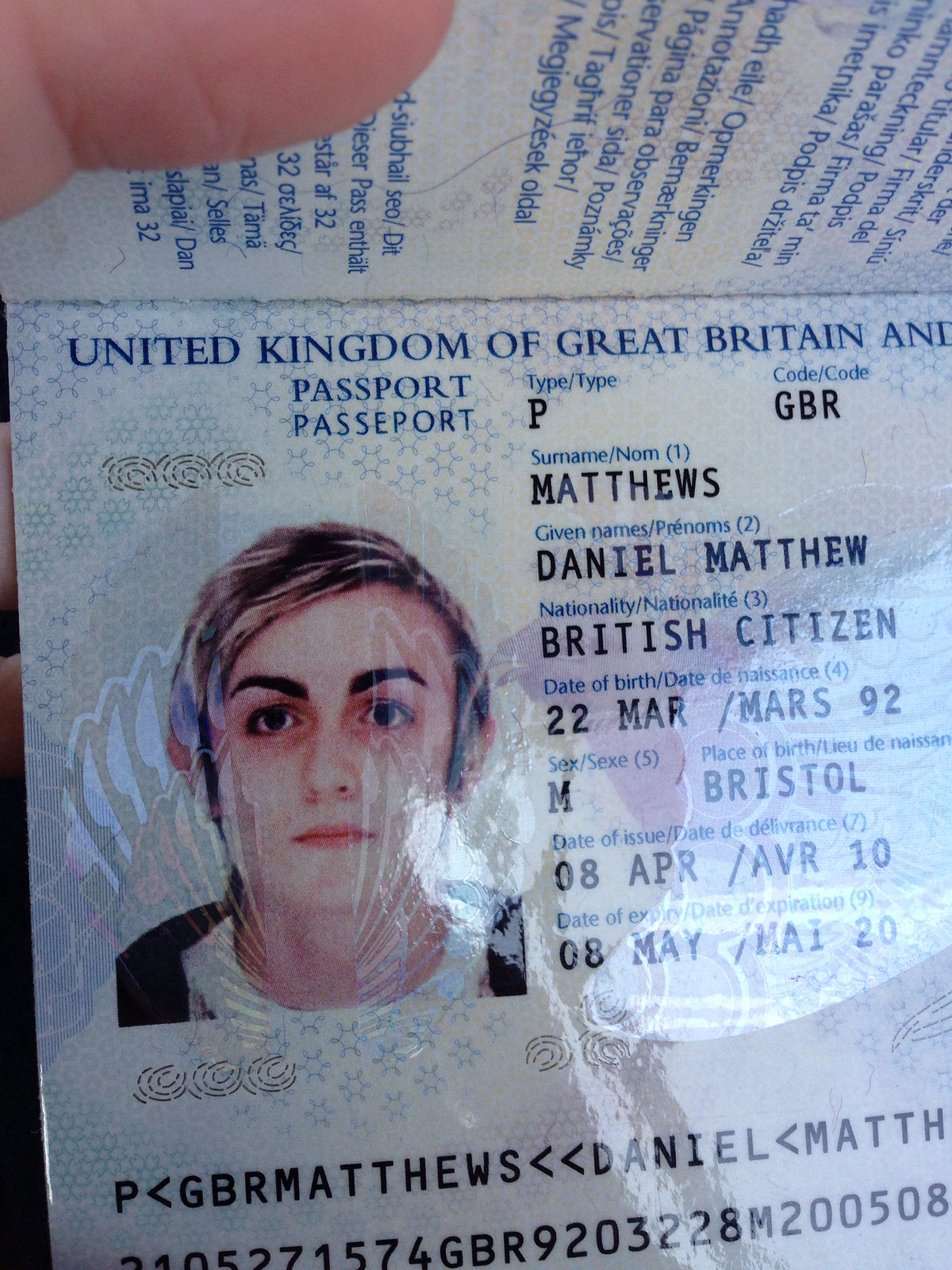This is a tall, vertically oriented image showing a close-up of the left side of an open passport. The seam of the passport is visible, running horizontally across the top, with a finger holding it open at the top left corner. The passport belongs to a young Caucasian male with short, blonde hair styled with frosted tips and thick brown eyebrows. He has notably red lips and is pictured against the left side of the passport.

At the top of the page, in blue font, it reads "United Kingdom of Great Britain," with "passport" written below. To the right of the photograph, several personal details are listed in black font: 

- Type: P
- Code: GBR
- Surname: Matthews
- Given Names: Daniel Matthew
- Nationality: British Citizen
- Date of Birth: 22 March 1992
- Sex: M
- Place of Birth: Bristol
- Date of Issue: 08 April 2010
- Date of Expiry: 08 May 2020

Below the photo, there is some computer-typed text that runs across the bottom of the page. This detailed close-up reveals the specific layout and important identifying details of the passport.